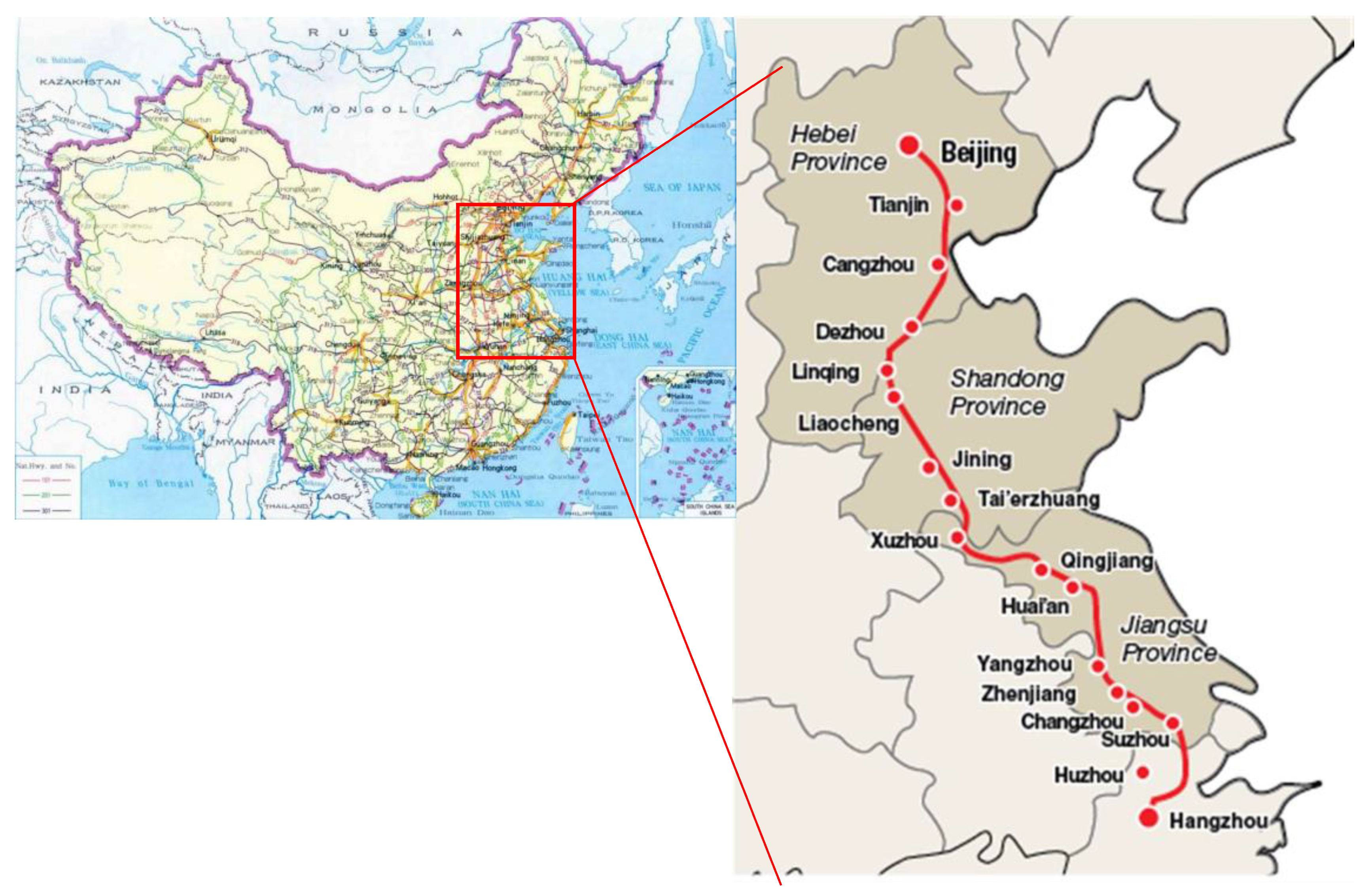The image features a two-part map of China. The smaller section on the left shows the entirety of China, colored in yellow with a purple outline, and surrounded by light blue oceans, including the Pacific Ocean. This segment highlights China's geographic position in Asia alongside neighboring countries such as India, Mongolia, and Russia. A red rectangular box highlights a region of central eastern China. 

From this boxed region, two red lines lead to a larger, zoomed-in portion on the right side of the image. This detailed map section extends roughly along the coast from Beijing in the north to Hangzhou in the south, tracing a red line that marks a road connecting several major cities. The zoomed-in map features the Hebei, Shandong, and Jiangsu provinces, illustrated in olive and tan hues with white seas. Key cities such as Beijing, Jinning, Huiyan, and Hangzhou are labeled and indicated by red points along the road. The maps use various colored lines to indicate major streets and thoroughfares, enhancing the clarity and navigability of the regions depicted.